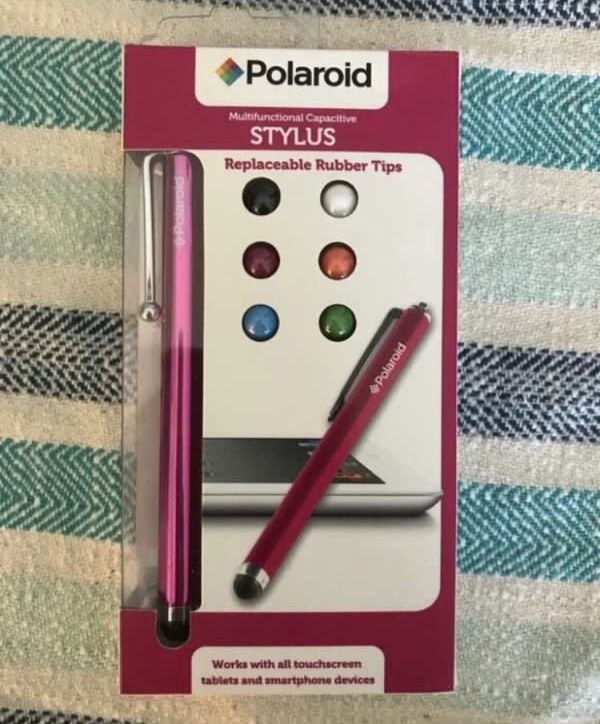This color photograph captures a large, prominently centered Polaroid Multifunctional Capacitive Stylus package set against a fabric with horizontal stripes in red, black, aqua, and white. The fabric background appears soft, resembling a blanket or tablecloth. The product is encased in a clear plastic package with a box design. The top section of the packaging has a purple-pink border with rounded white rectangular background featuring the black text "Polaroid." Below this, in a pink area, it reads "Multifunctional Capacitive Stylus." Inside the transparent middle section, a pink stylus with a chrome pocket clip is visible. To the right of the stylus, on a white background, six multicolored dots represent replaceable rubber tips, with the text "Replaceable Rubber Tips" in red above them. An image of a smartphone or tablet is also visible on the packaging. At the bottom, another white section declares in black text, "Works with all touch screens, tablets, and smartphone devices."